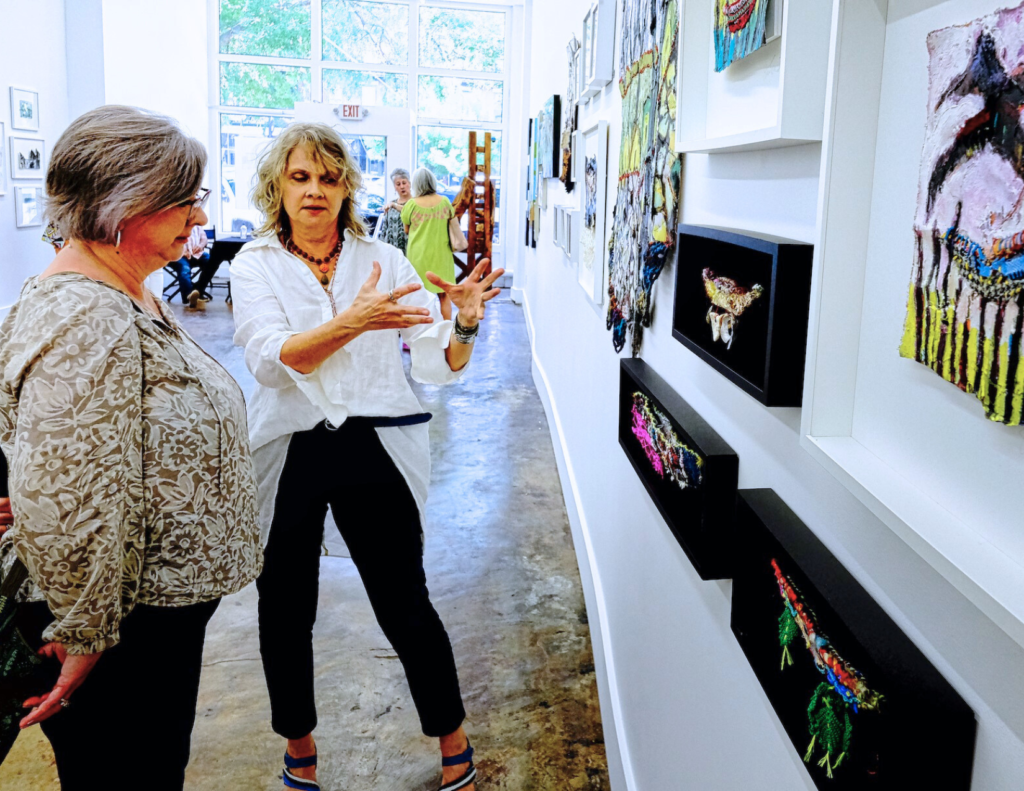This photograph captures a lively scene in a gallery or store specializing in art and handmade items. At the forefront, two women are engaged in animated conversation in front of two horizontal black shadow boxes that display brightly colored necklaces. The woman on the left, who is perhaps in her 60s, has grayish-brown hair and wears glasses. She is dressed in a green shirt decorated with a white floral motif and black pants. To her right, the woman enthusiastically explaining the artwork is about 50 years old. She has blondish-brown hair and dons a dark brown beaded necklace. Her oversized white button-down shirt, rolled up to her elbows, is tucked into her black ankle-length pants, and she completes her outfit with black strap sandals. The speaker elaborates on the artwork with expressive hand gestures. In the background, two more women can be seen. The store’s white walls are adorned with various pieces of art that stretch down the hallway, shrinking into the distance.